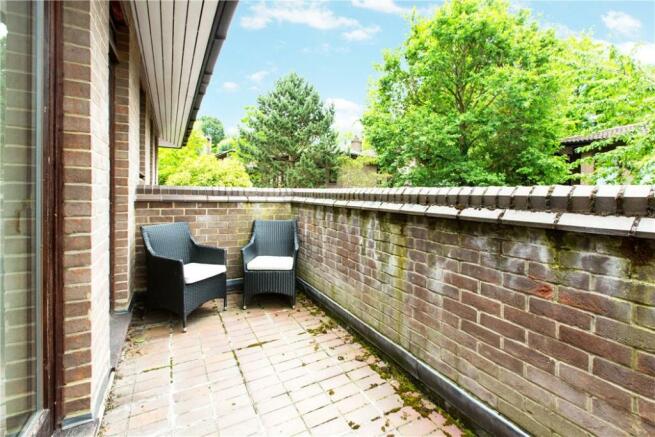This image depicts an outdoor balcony or patio area on what appears to be someone's apartment. The setting features red brick walls and flooring, with an overhang of white wood that extends a few feet above, not covering the entire area. The brick walls rise to about waist height. On the left side, there are sliding glass patio doors beneath the overhang, with windows adjacent to them. Positioned towards the back left of the balcony are two dark gray wicker chairs, each adorned with light-colored cushions, possibly white. The chairs have high arms and appear comfortable for seating. In the background, verdant, well-tended trees can be seen against a backdrop of a clear blue sky with only a few white clouds. The trees are lush and healthy, indicating good care. Additionally, to the right, there is a partial view of the roof of another building, similar in color to the balcony's bricks.